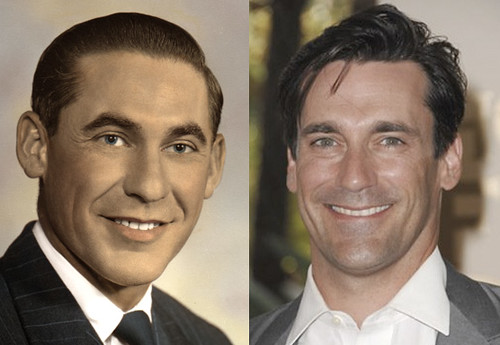The image features two closely-cropped photographs placed side by side. On the right is John Ham, who is smiling and revealing the top row of his teeth. He has slightly messy brown hair that is mostly brushed back, with a few strands falling onto his forehead. John is wearing a light and medium gray suit with a white button-up shirt underneath. His eyes are light blue.

On the left is another man, also smiling and showing the top row of his teeth. He has slicked-back, dark brown hair and slightly darker light blue eyes compared to John. He is dressed in a black jacket with white stripes, a matching dark gray tie, and a white collared shirt. The background behind him is a solid beige color, contrasting with the more dynamic backdrop behind John, which appears to feature forest-themed billboards.